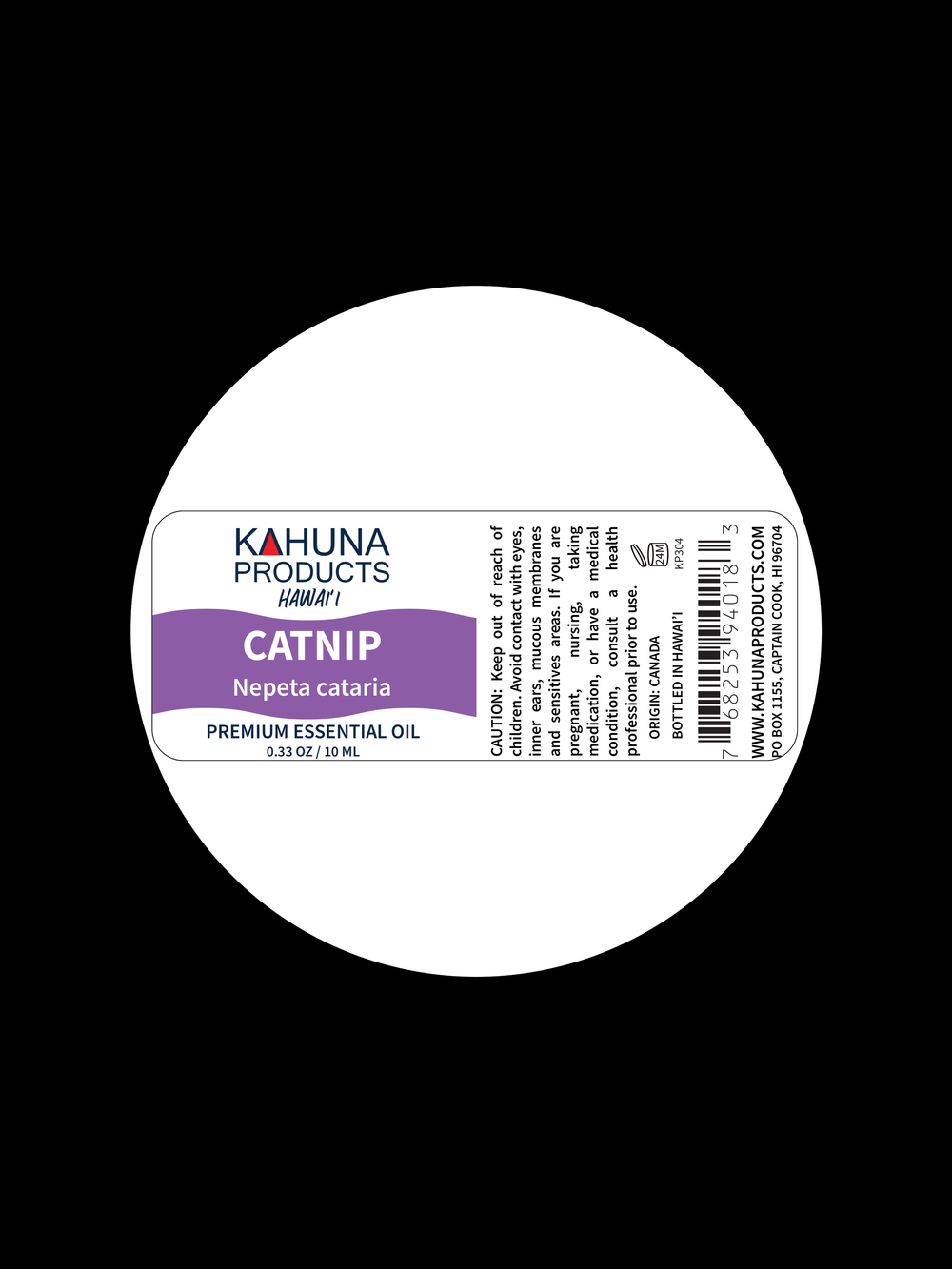The product image features a sleek, all-black background with a prominent white circle in the center. A rectangular label with rounded top corners is placed within this circle, divided into two sections. On the left side, the label introduces "Kahuna Products Hawaii" in black text at the top, followed by a purple banner that reads "Catnip Nepeta Cataria" in white. Below this, it states "Premium Essential Oil" and specifies the quantity as "0.33 ounces" or "10 ml" in black text. The right side of the label includes various details: a caution warning, barcode, website (kahunaproducts.com), and the product’s origin and bottling information, which notes that the oil originates from Canada and is bottled in Hawaii. Additionally, it carries detailed usage warnings, advising to keep the product out of children's reach, avoid contact with eyes, inner ears, mucous membranes, and sensitive areas, and to consult a health professional if pregnant, nursing, taking medication, or having a medical condition.